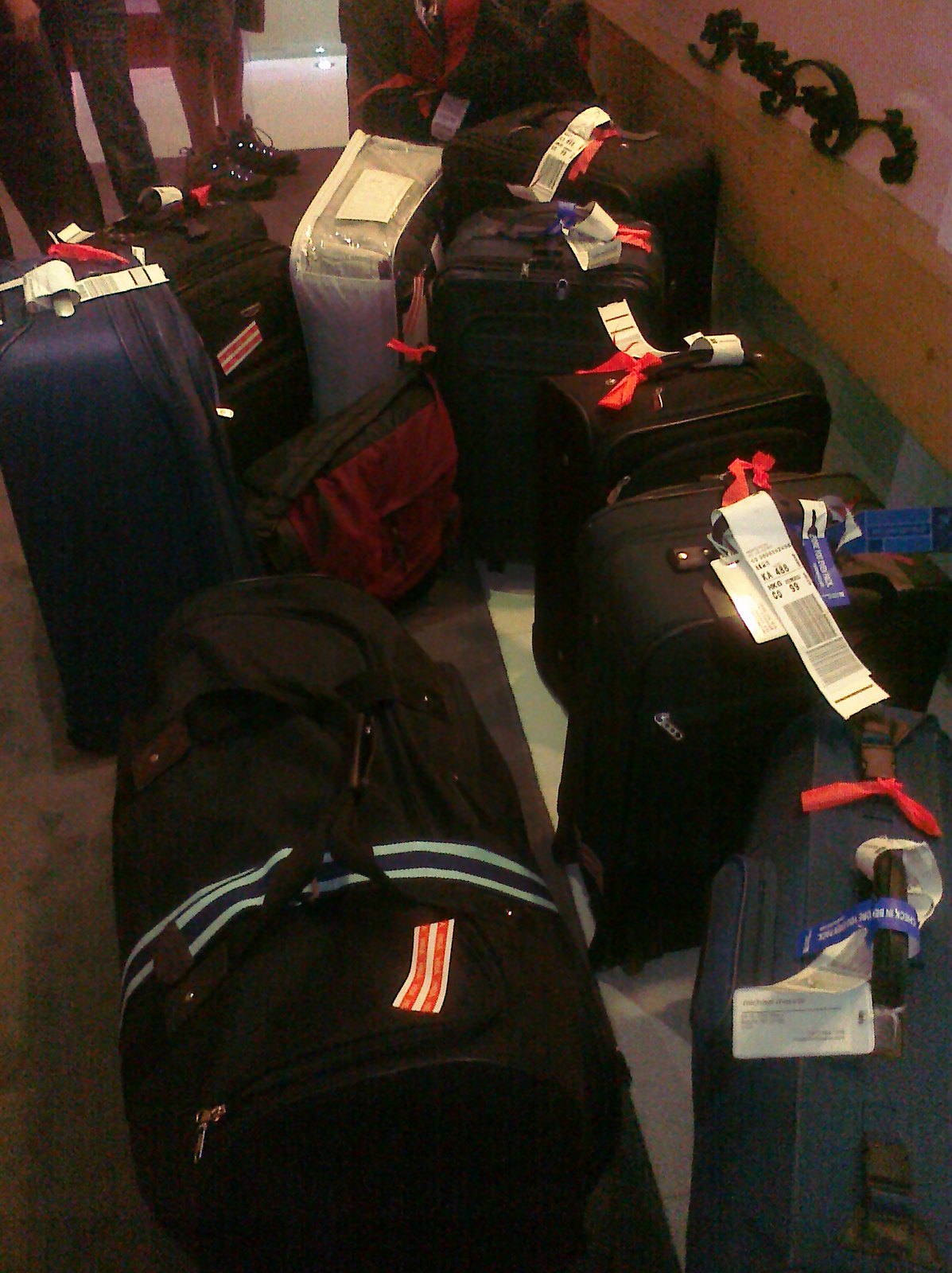The image depicts a chaotic array of luggage in a hallway. There are around 10 large suitcases and travel bags, primarily black with a few dark blue, a red backpack, and a light gray suitcase. The suitcases feature red or red-orange ribbon tags and white airline stickers on the handles. There's a prominent black duffel bag in the foreground and a navy blue suitcase to its right. The floor is divided into a black and light brown rug extending into the background and a light gray section on the right. On the right wall, a small wooden shelf is situated above a green-painted lower portion, with black text or artwork above the shelf. In the background, partially obscured, are people's legs and feet, suggesting they are checking in or waiting in a busy space, possibly a hotel or an airport.